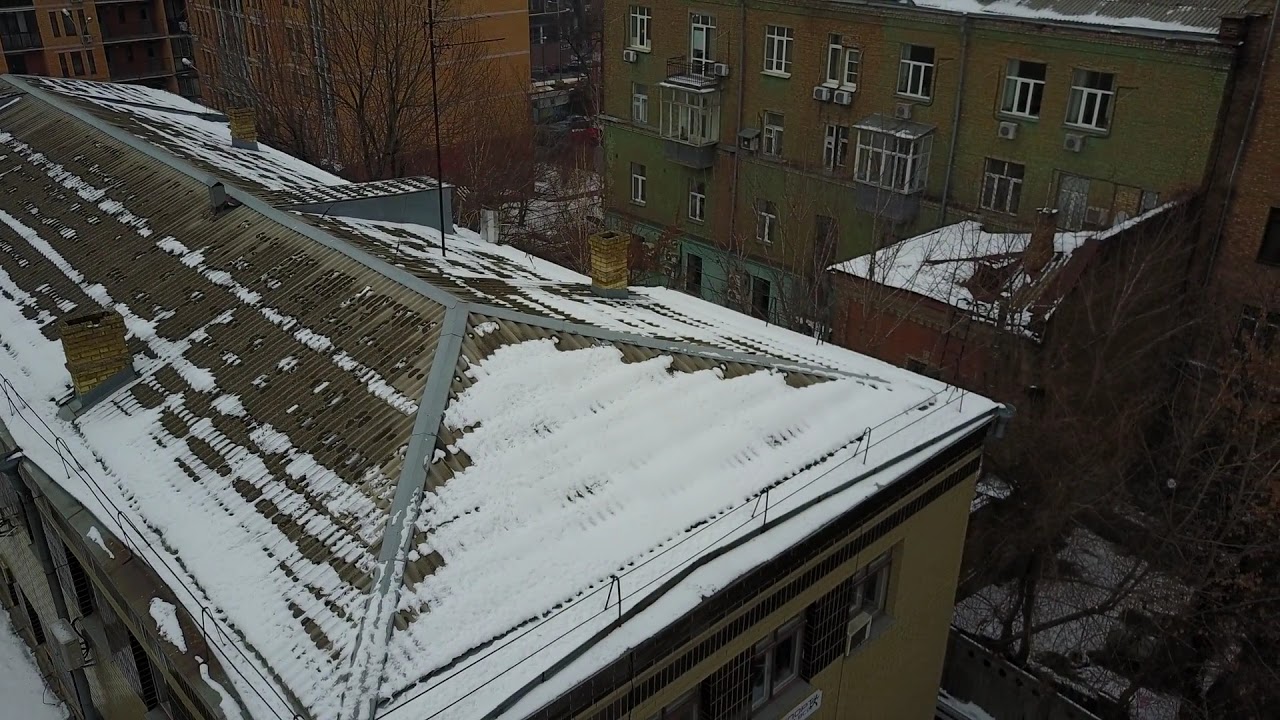This aerial photograph captures the roof of a long building, which appears to be a complex of four interconnected residential homes. The roof, partially covered with a light dusting of snow that reveals brown patches, suggests an autumn or early winter setting. Spread across the roof are several chimneys. The background features two taller adjacent buildings; one is a four-story structure with a gray-green exterior and rows of windows, and the other is an orangish-brown brick building. Surrounding the buildings are numerous trees with bare branches, indicating the season. The photo, likely taken in a metropolitan city from a high vantage point or by a drone, presents a dark, industrial ambiance reminiscent of an East Coast city. The lack of visible people or cars and the cloudy daytime sky also contribute to the scene's tranquil and somewhat somber atmosphere.